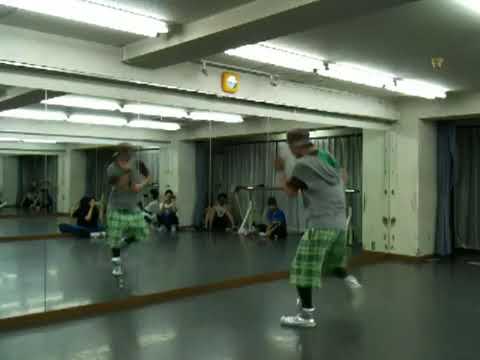In this detailed indoor image, a young man is dancing in what appears to be a hip-hop dance studio, which features a wall completely covered with large mirrors. He is captured mid-movement, balancing on one leg with the other lifted in the air. His outfit consists of a gray short-sleeved hoodie with a black shirt underneath, green plaid shorts, black socks, white sneakers, and a backward gray hat. The dance studio has a striking gray shiny floor and white ceiling adorned with long strips of white lights. Reflecting in the mirror, four other young men are seen sitting on the floor, intently watching the dancer, possibly as part of a dance lesson. Additionally, gray curtains are visible in the background, drawn shut to perhaps control the lighting provided by the indoor electric lights.